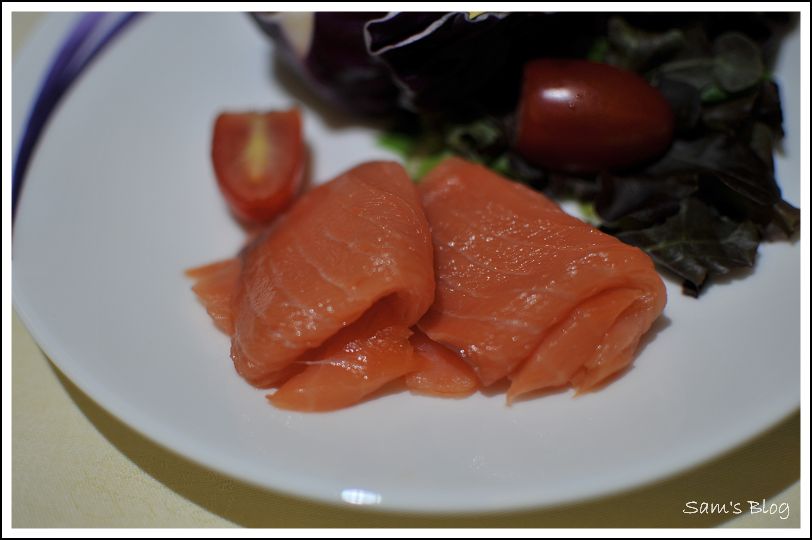This close-up photograph captures a carefully arranged plate of food on a plain white, circular porcelain plate. In the foreground and occupying the center stage of the composition are thinly sliced pieces of raw salmon, artfully folded into curves, emphasizing their pinkish-orange hue. Directly behind the salmon lies a fresh salad made of dark leafy lettuce and cherry tomatoes—the deep red of the tomatoes contrasting with the green leaves. One of the cherry tomatoes is whole while another is neatly cut in half. Although the background of the image is blurred, a blue arc is discernible in the upper left-hand corner. Notably, the lower right-hand corner features the watermark, "Sam's Blog," in white text. The plate rests on a cream-colored or yellow surface, casting a discernible shadow towards the viewer. This image appears to be professionally styled, possibly for a culinary blog or a social media post dedicated to food photography.